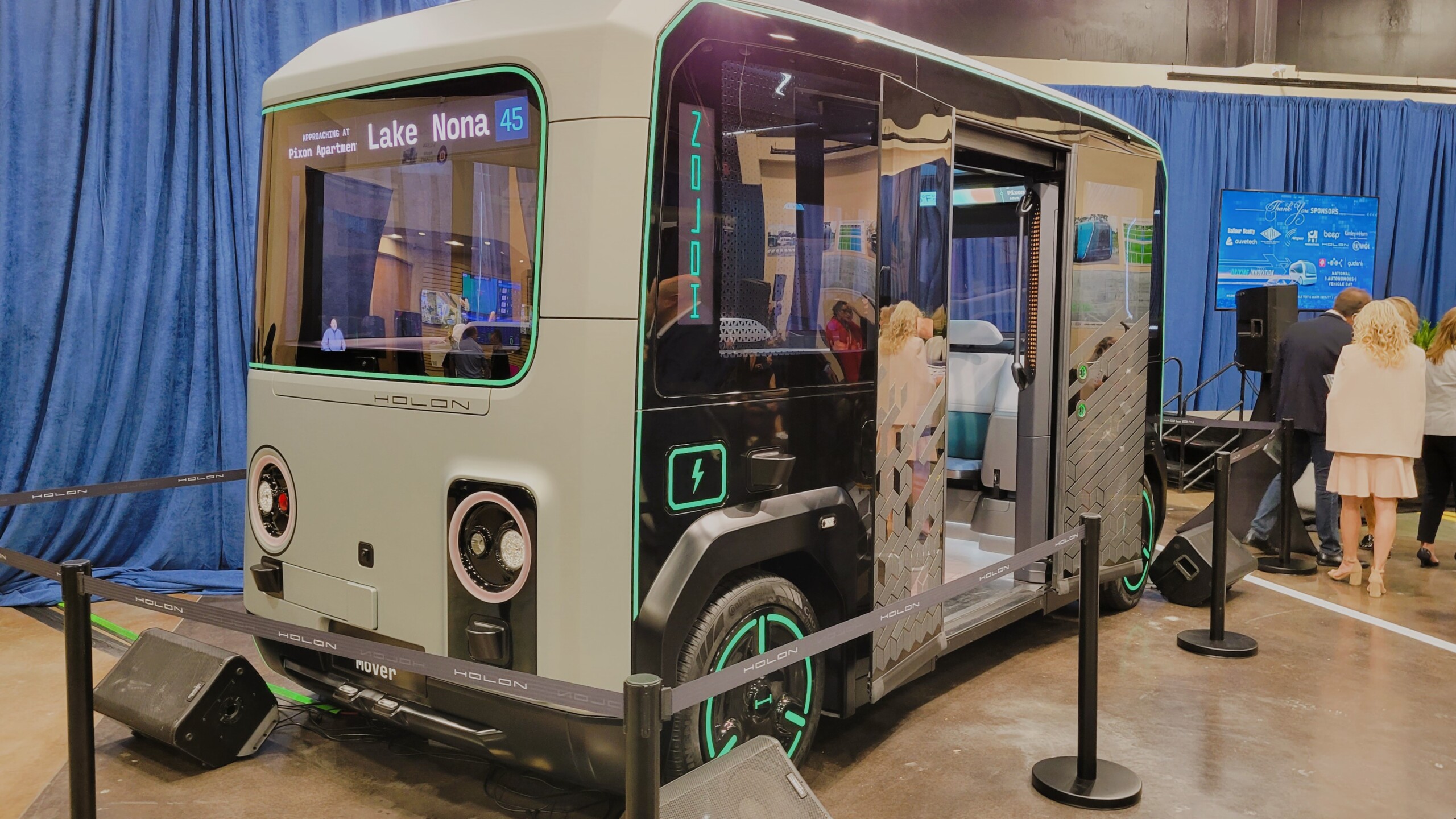This photograph captures a small, electric mini bus displayed at an exhibition, potentially focused on green technology or automotive innovations. The vehicle, most likely produced by Holden, exhibits a slightly futuristic aesthetic, suggesting it might not yet be a common sight on the streets. Positioned on a wooden floor, the bus is cordoned off with black ropes connected to black poles. The mini bus has a distinctive flat-faced front with two large, round headlights on the lower left corner and a prominent rectangular front window. The door is open, revealing a white seat and a small blue table inside.

Adorned in green, the bus includes an electric symbol located above its left wheel, which is black with a greenish light ring on the inside. The vehicle has small, stylized details like an electric symbol and a black bar on top with the text "Lake Nona 45" on the right, although additional text to the left of this is not legible. Surrounding the bus are blue curtains and a black wall above. 

To the right of the vehicle, a group of people—two men and two women—are gathered around what appears to be a stage or table, indicating part of a broader presentation or discussion. The bus itself has a sliding door, hinting at its practical design for easy access, and the interior window is accentuated with a green outline, harmonizing with its eco-friendly theme. This vehicle, possibly intended for camping or short trips, showcases innovative green technology in a compact form.